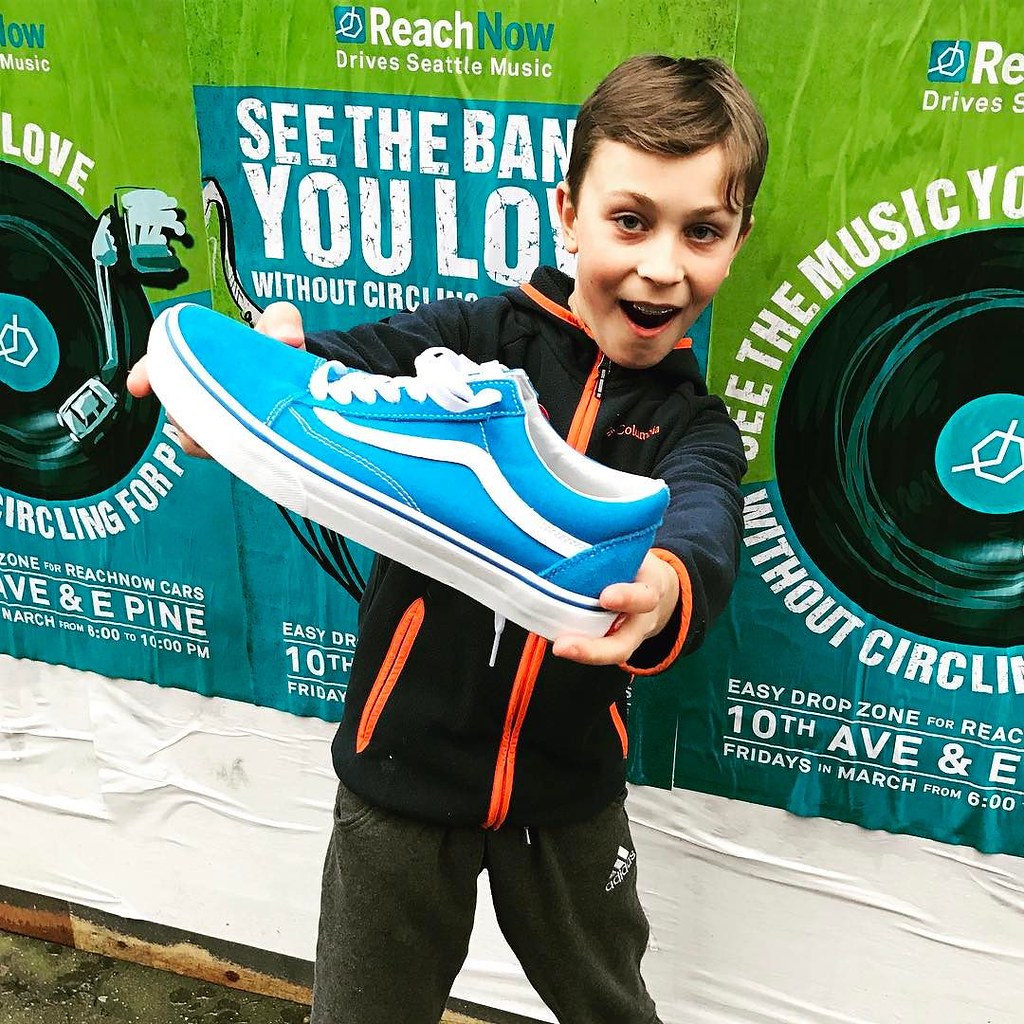In the photorealistic image, a young boy with brown hair and braces looks directly into the camera, his mouth open as if speaking or expressing surprise. He is holding up a large, bright blue sneaker with a white sole, white laces, and a central white stripe running from the end of the laces to the heel. The child is dressed in a black jacket with an orange zipper and pockets, paired with brown Adidas pants. Behind him, a series of green and blue posters can be seen, featuring stylized black and blue records and adorned with white text. The text includes phrases like "REACH NOW," "DRIVE," "SEATTLE MUSIC," "10th AVENUE," "EASY DROP ZONE," "FRIDAYS IN MARCH," and "JUNE 6TH." A white platform is also visible directly behind the boy, who appears to be showcasing the blue sneaker prominently for the camera.